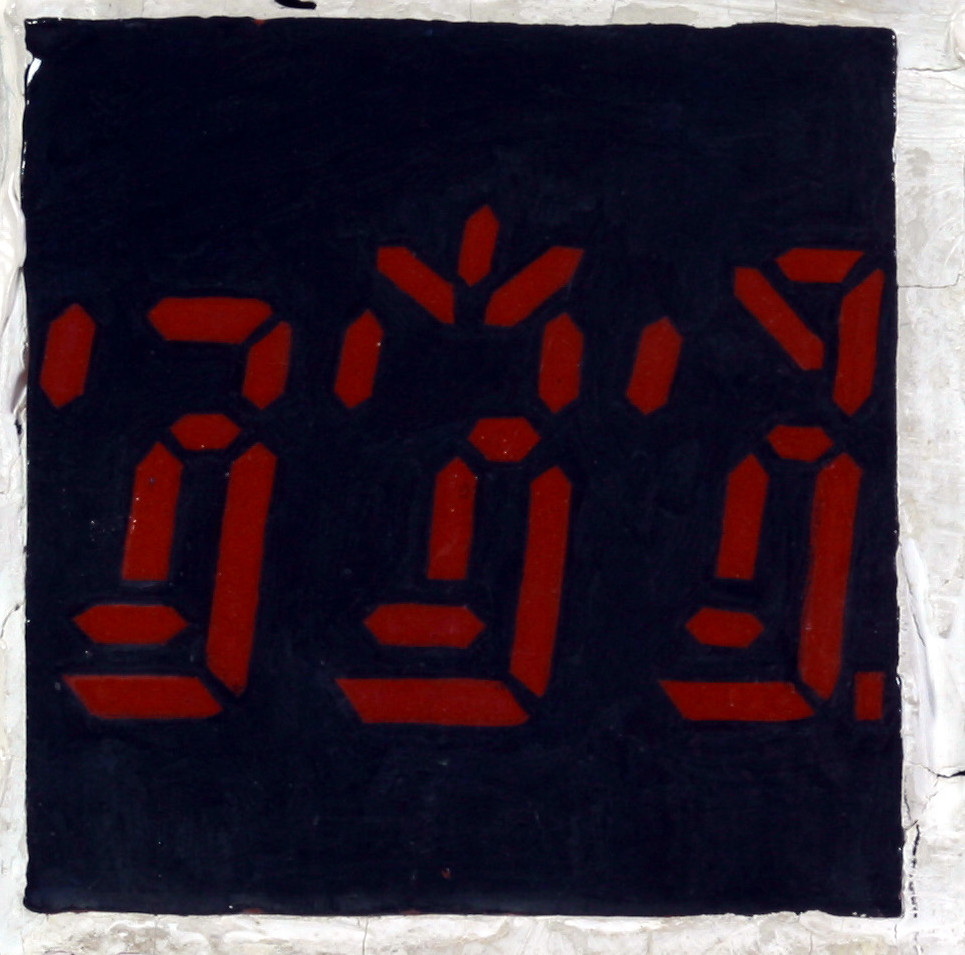The image depicts a sign on a white brick wall, which is cracked and worn, particularly on the bottom right. The central element of the image is a black square or rectangular frame, possibly a print or painted canvas, set against this white background. Inside this black frame, there are three distinct red symbols or letters, arranged horizontally. The symbols appear somewhat angular and digital-like in style, with the first resembling a "3", the second a "3" with a crown-like top, and the third a stylized "J" with a pointed end at the top. The red symbols contrast sharply with the black background, making them stand out prominently despite their ambiguous and foreign nature.